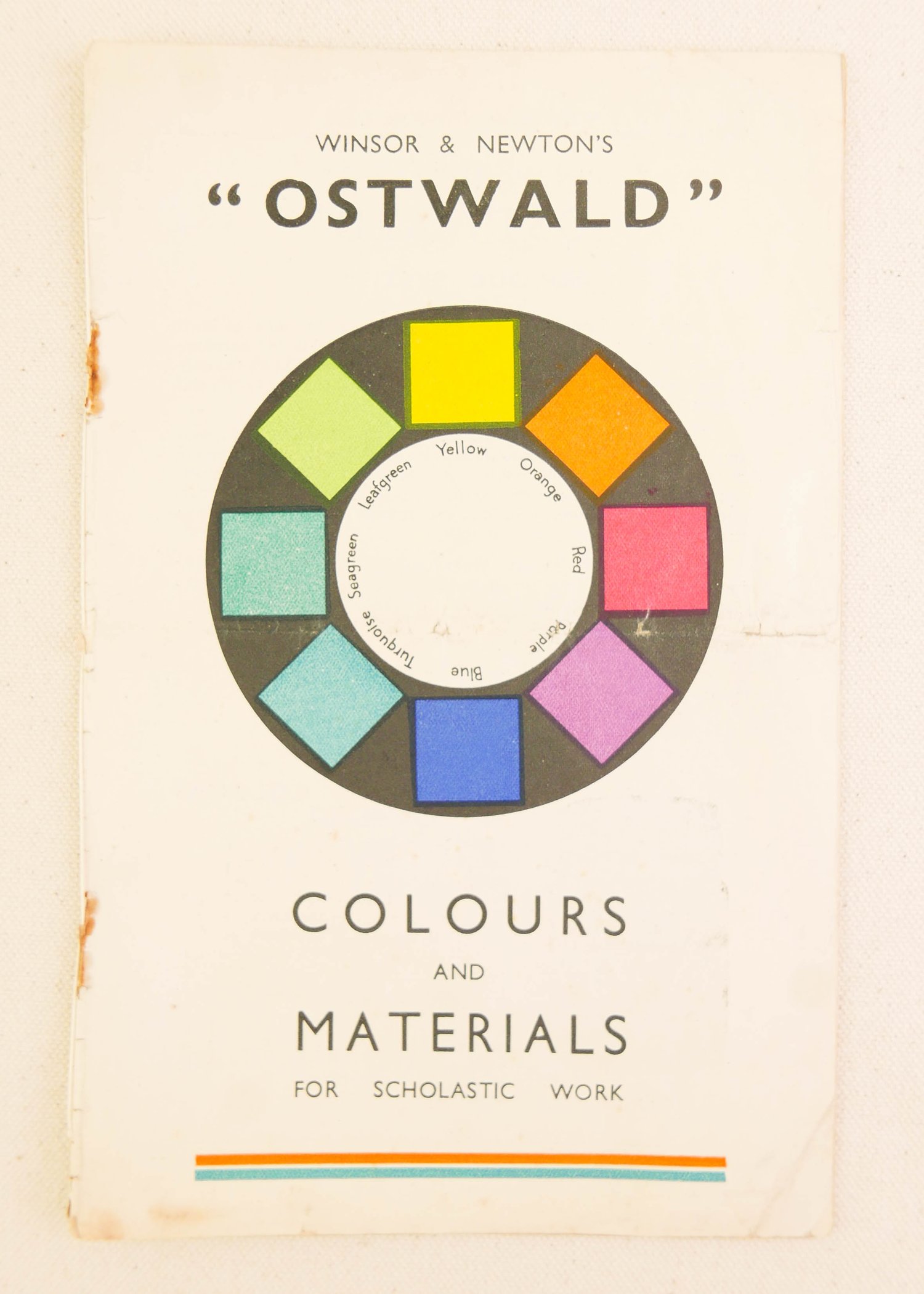The photograph captures the aged cover of a book or pamphlet, presenting a vintage appearance with slightly beat-up, off-white eggshell pages. Notably, there are two distinct orange rust marks, likely from staples in the binding, located towards the top and bottom on the left side of the cover. Additionally, some grease-like orange-red marks are evident in the bottom left corner. 

Prominently, the top of the cover features the title in a very dark gray, almost black font, presented in all caps: "WINDSOR AND NEWTON'S." Beneath this, in a larger and bolder font and surrounded by double quotation marks, is the name "OSTWALD". 

At the center of the cover, a detailed color wheel stands out. This wheel includes a brown outer circle encasing eight different colored squares, each labeled with their respective colors: yellow, orange, red, purple, blue, turquoise, sea green, and leaf green. Inside the brown circle is a white circle. Below the color wheel, the text in the same dark gray font reads, "COLORS AND MATERIALS FOR SCHOLASTIC WORK." The cover's background shares the same creamy tone as the paper, adding to its antique look with smudges and additional marks hinting at its age and use.